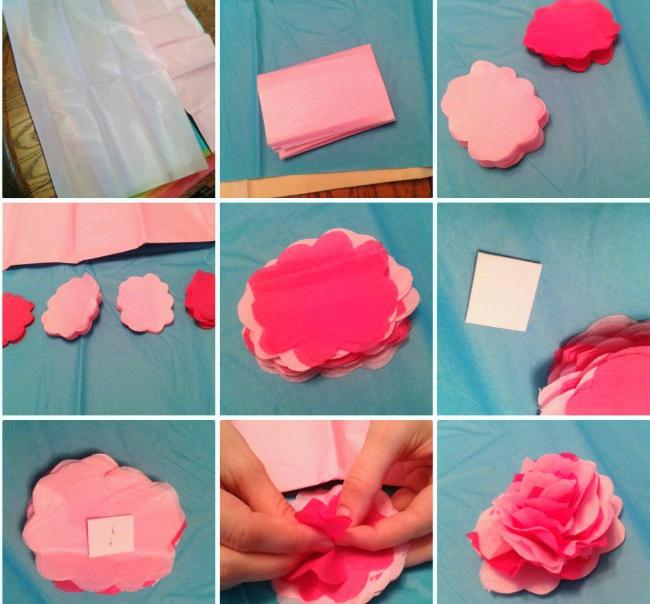This collage of nine images meticulously demonstrates the step-by-step process of creating a fabric flower, although the material could be some kind of paper product. The sequence begins in the top left with sheets of paper or plastic on a wooden table. By the second image, the material is placed on a teal-colored tablecloth, seen throughout the remaining images. 

The initial step displays square sheets of pink material. These sheets are cut into flower-like shapes with alternating light pink and dark pink hues in subsequent images. As the process progresses, the fourth and fifth images reveal rows of these petal shapes, precisely positioned and layered in an alternating pattern.

Mid-sequence, a small white piece of paper appears, which gets stapled to the back of the layered petals in the sixth and seventh images. The eighth image captures the intricate bending and twisting of these layers to fashion the petals realistically. Finally, the bottom right image showcases the complete, intricately crafted fabric flower.

The collage, devoid of textual instructions, visually guides the viewer through the creative construction of a colorful, delicate flower, effectively using the contrasting hues of pink against the teal cloth background and emphasizing hands-on crafting steps.